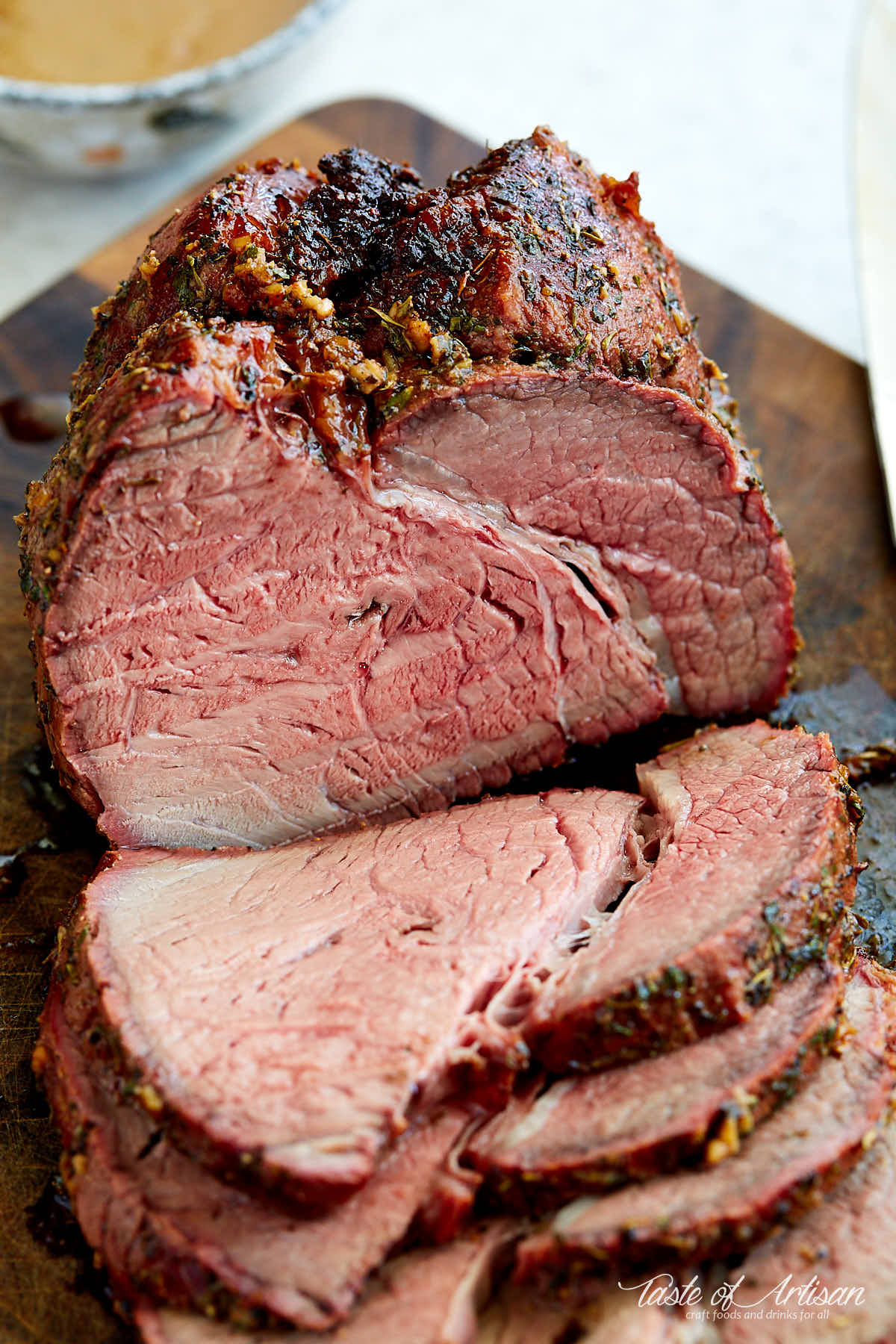This is a professionally taken, color photograph of a delectable roast, possibly beef, displayed in portrait orientation. The roast is beautifully cooked and sits on a dark wooden cutting board, positioned on a white countertop. The meat has a well-seasoned, browned, and slightly charred crust, indicating a mix of herbs and spices, with some potential hints of green and orange seasoning visible on the crust. The interior is cooked to a medium rare, showcasing a pinkish-red color marbled with some white fat. Several thin slices of the roast—approximately four—have been cut and are stacked neatly towards the bottom of the image, revealing the juicy and tender inside of the meat.

In the background, softly blurred, there's a white bowl containing a yellowy or brownish substance, possibly a soup or sauce, adding a complementary touch to the visual presentation. At the bottom of the image, white cursive lettering reads, "Taste of Artisan, craft foods and drinks for all," giving the impression of a high-end food advertisement.